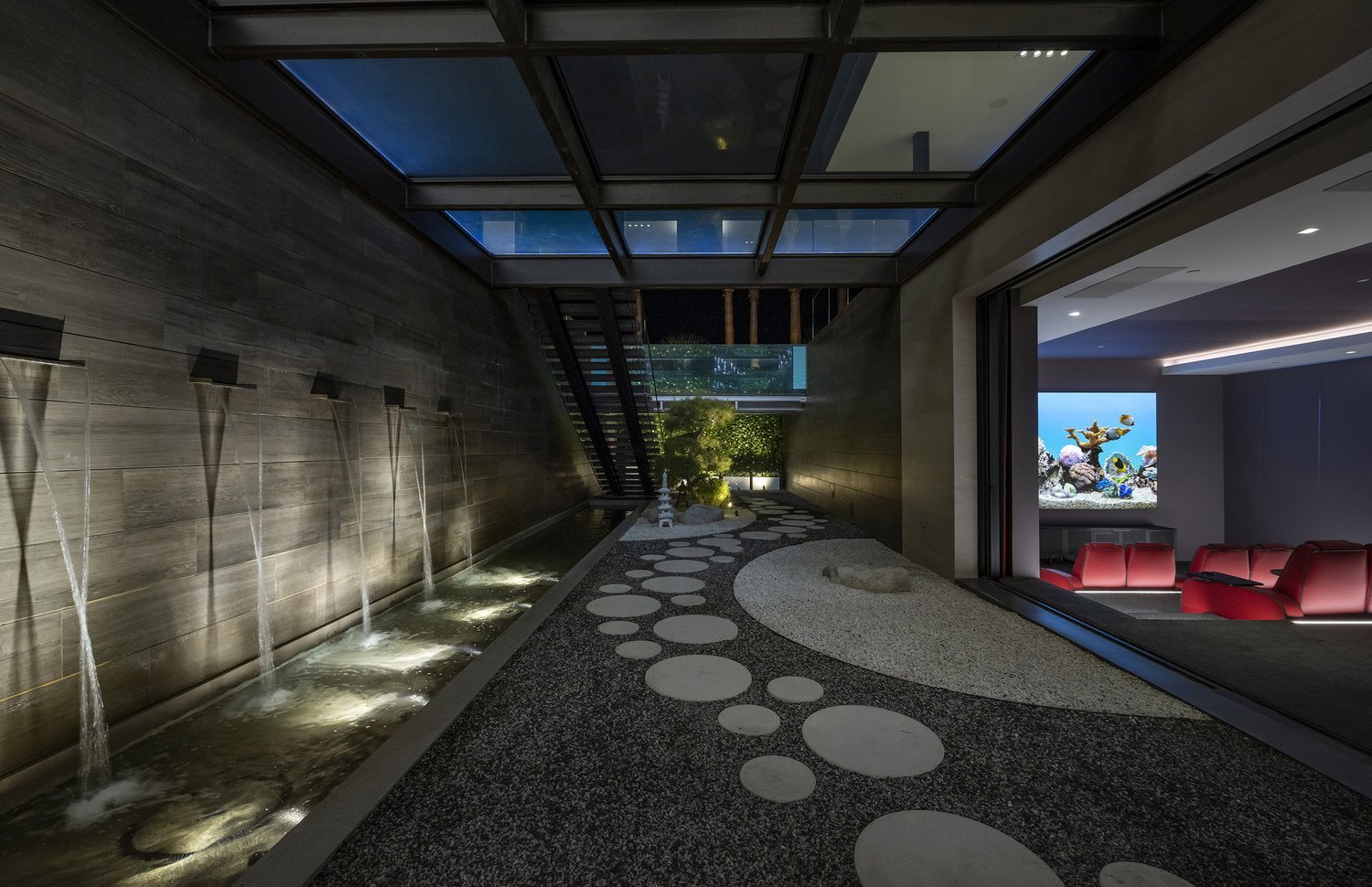The image depicts an opulent, high-end hallway within a mansion, designed with extraordinary attention to luxury and detail. On the right side of the dimly lit hallway, there's an extravagant home movie theater featuring red, paired chairs, separated by spaces, all facing a screen that displays a fish aquarium, adding a touch of serenity. The theater area, encapsulated by a gray, modern design, gives off an aura of lavishness and sophistication. Adjacent to this, a large glass wall or opening accentuates the grandeur of the space.

To the left of the hallway, there's a long, narrow, rectangular pool into which water fountains cascade from a stone wall, contributing to a meditative, Japanese-inspired ambiance. The walkway itself is adorned with circular carpeting or stone steps, enhancing the tranquil and meticulous aesthetic. In the background, a glass-floored staircase ascends, further emphasizing the luxurious and expansive nature of this high-end residence.